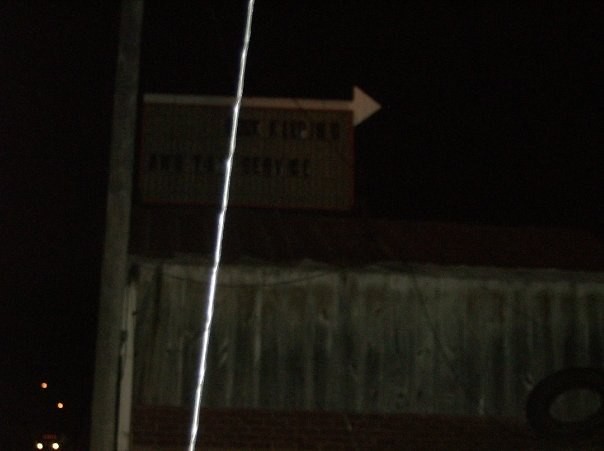This image, taken at night, depicts a side of a red brick building obscured by darkness. The overall appearance is quite blurry and low-resolution, adding to the fuzzy, indistinct quality of the scene. On the upper portion of the building, there's a rectangular yellow sign with unreadable black text, crowned by a right-pointing white arrow. Below this sign, dark gray windows with a white outline are visible, though some are boarded up or covered in translucent plastic. In the bottom left corner of the image, the piercing glow of four distant car headlights—white and orange—punctuates the darkness. A vertical white wire dangles prominently in the foreground, clashing starkly against the shadowy backdrop of the building. A wooden pole runs along the left edge, adding to the vertical elements in this low-light, atmospheric capture.